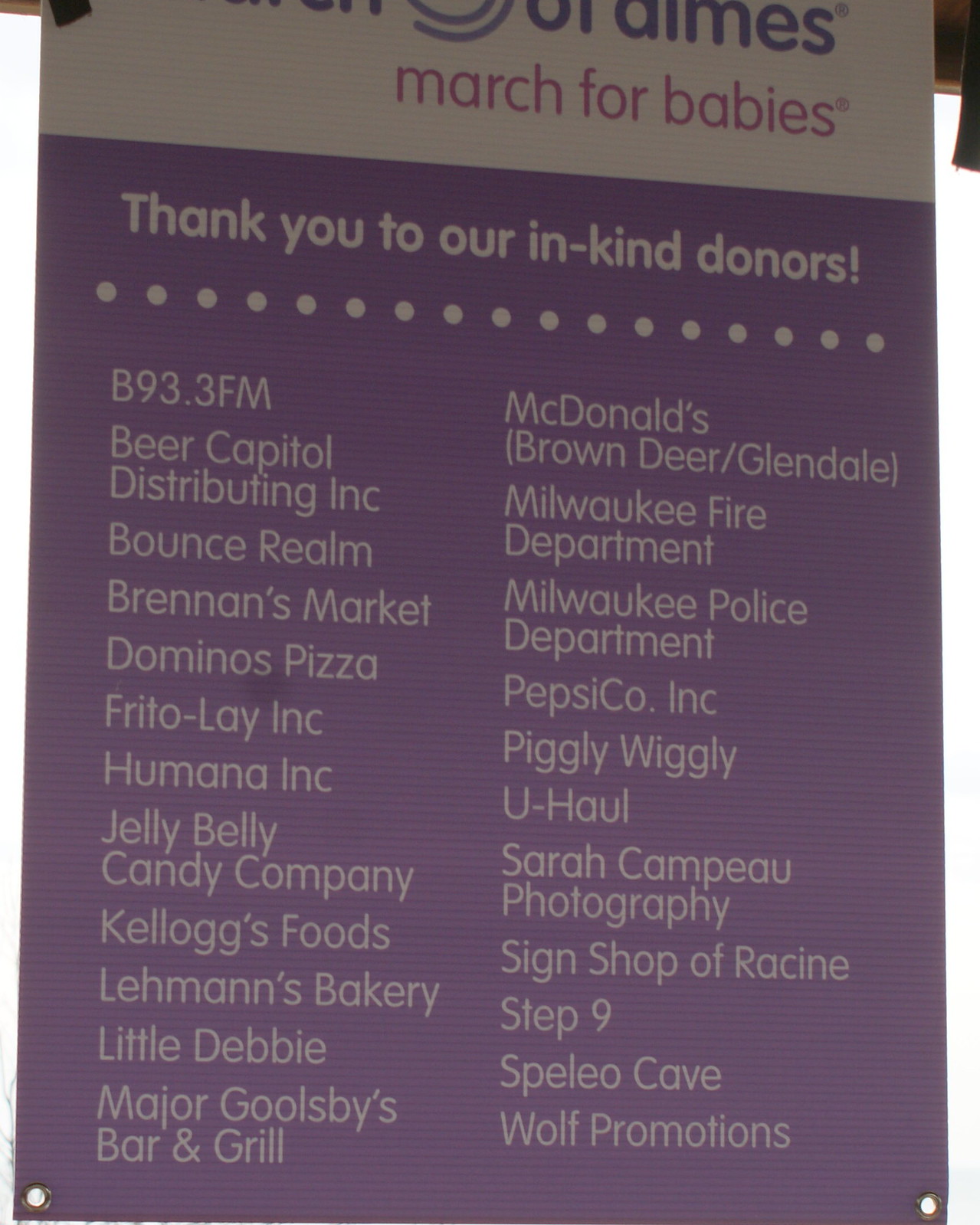The image depicts a large, partially obscured sign or banner, thanking donors affiliated with the March of Dimes' "March for Babies" event. The top half of the sign is white and features the "March for Babies" and "March of Dimes" logos, though the text is slightly cut off. The lower half of the sign transitions to a light purple background with white text that reads, "Thank you to our in-kind donors." The list of donors appears in two columns, presented in a light cream color against the purple backdrop. Notable donors include:

- B93.3 FM
- Beer Capital Distributing, Inc.
- Bounce Realm
- Brennan's Market
- Domino's Pizza
- Frito-Lay, Inc.
- Humana, Inc.
- Jelly Belly Candy Company
- Kellogg's Foods
- Lehman's Bakery
- Little Debbie
- Major Goolsby's Bar and Grill
- McDonald's
- Brown Deer
- Glendale
- Milwaukee Fire Department
- Milwaukee Police Department
- PepsiCo, Inc.
- Piggly Wiggly
- U-Haul
- Sarah Campo Photography
- Sign Shop of Racine
- Step Nine
- Speleo Cave
- Wolf Promotions